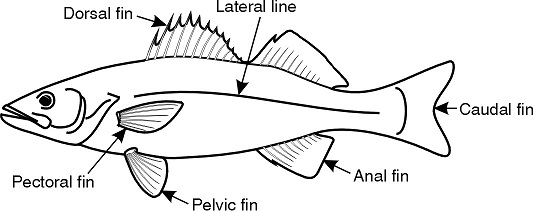The image depicts a detailed, black-and-white illustration of a streamlined game fish, resembling a salmon or trout, with several anatomical features labeled. The fish is oriented to the left, outlined in dark black against a white background. Key parts are marked with arrows and labels in black font: the dorsal fin at the top, the lateral line running along the body’s center, the caudal fin at the tail, the anal fin on the underside near the tail, the pelvic fin below the midsection behind the gills, and the pectoral fin just below the gills. The fish has distinguishing features like a white body with light black lines on the fins, open mouth, and visible eye. The illustration serves as an educational chart of fish anatomy.